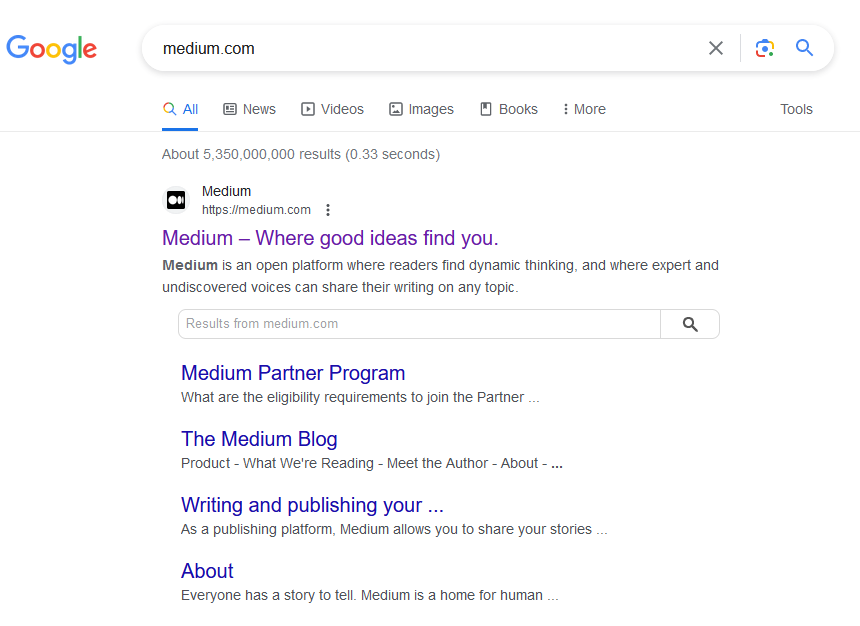The image is a detailed screenshot of Google search results on a white background. The iconic Google logo, with its letters in vibrant colors, is prominently displayed in the top left corner. Below the logo is a long search bar that spans nearly the entire width of the page, with the phrase "medium.com" entered into it.

Beneath the search bar are several tabs including "All," "News," "Videos," "Images," "Books," "More," and "Tools," with the "All" tab selected. The search indicates approximately 5,350,000,000 results. The top search result is for "Medium," located at medium.com, accompanied by a brief description: "Medium: Where good ideas find you. Medium is an open platform for readers to find dynamic thinking and where expert and undiscovered voices can share their writing on any topic."

Following this is another search bar labeled "Results from medium.com," with a magnifying glass icon on the far right. Below this bar are four specific search results within the medium.com domain:

1. **Medium Partner Program:** An article detailing the eligibility requirements to join the Medium Partner Program.
2. **The Medium Blog:** Topics include product updates, what the Medium team is reading, meet the author segments, and more.
3. **Writing and Publishing:** This result describes Medium's functionality as a publishing platform, allowing users to share their stories.
4. **About Medium:** An overview stating that everyone has a story to tell and that Medium is a home for human stories.